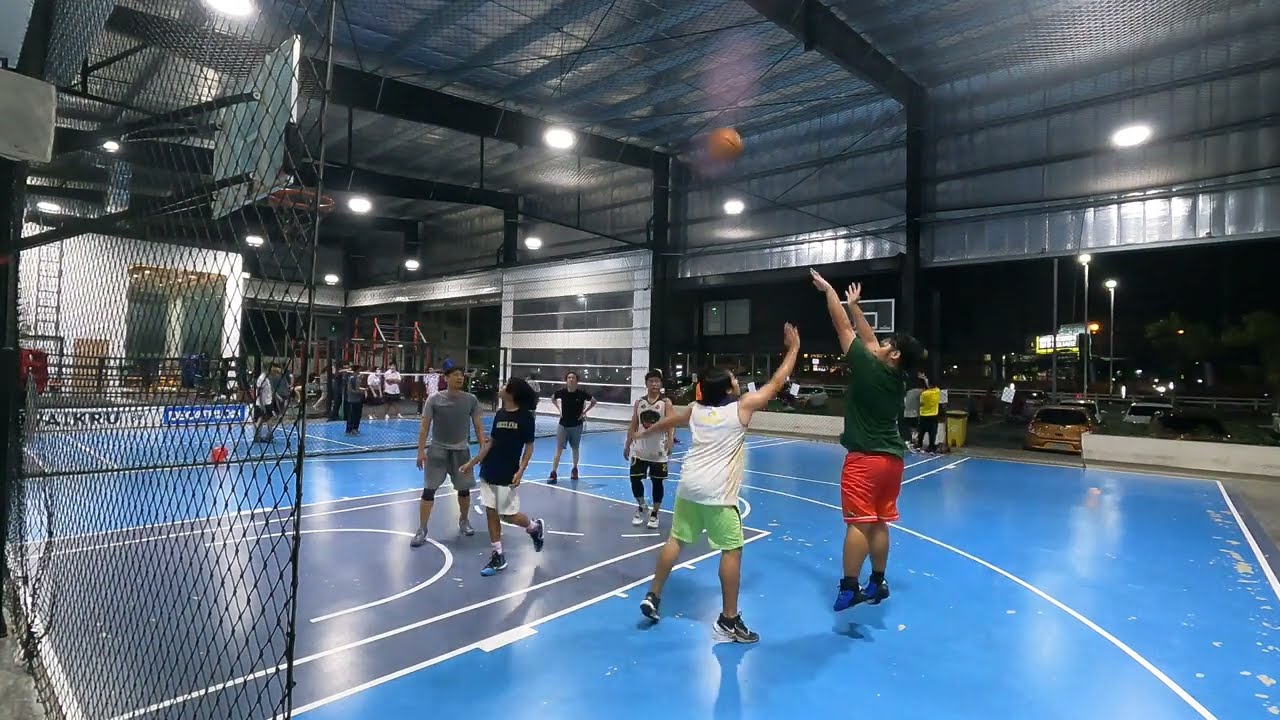In an expansive indoor gym with a roof reaching 20-30 feet high and featuring exposed beams, a lively basketball game unfolds. The structure resembles a metal Quonset hut, with one side open to the dark evening sky, revealing cars in a nearby parking lot. This hybrid indoor-outdoor space has no traditional walls or doors, adding to its unique atmosphere. The neon blue court, painted a striking bright hue, stands out vividly. In the left foreground, a wire mesh backstop and basket frame a rectangular gray free throw zone. 

At the focus of the scene is a dynamic moment: a young player in red shorts, blue shoes, and a black shirt is airborne, poised to take a three-point shot. Opposing them is another player in green shorts and a white sleeveless shirt, ready to block the shot, wearing Nike sneakers. The scene captures the essence of a casual pickup game, with players in various colorful attire.

Beyond the main court, other recreational areas are visible—a volleyball court and a boxing ring hint at the gym's multipurpose nature. Another basketball court adjacent hosts more players, emphasizing the facility's vibrant, communal atmosphere. The blue courts, in varying shades, dominate the view, anchoring the lively activity within this spacious, unconventional gym.